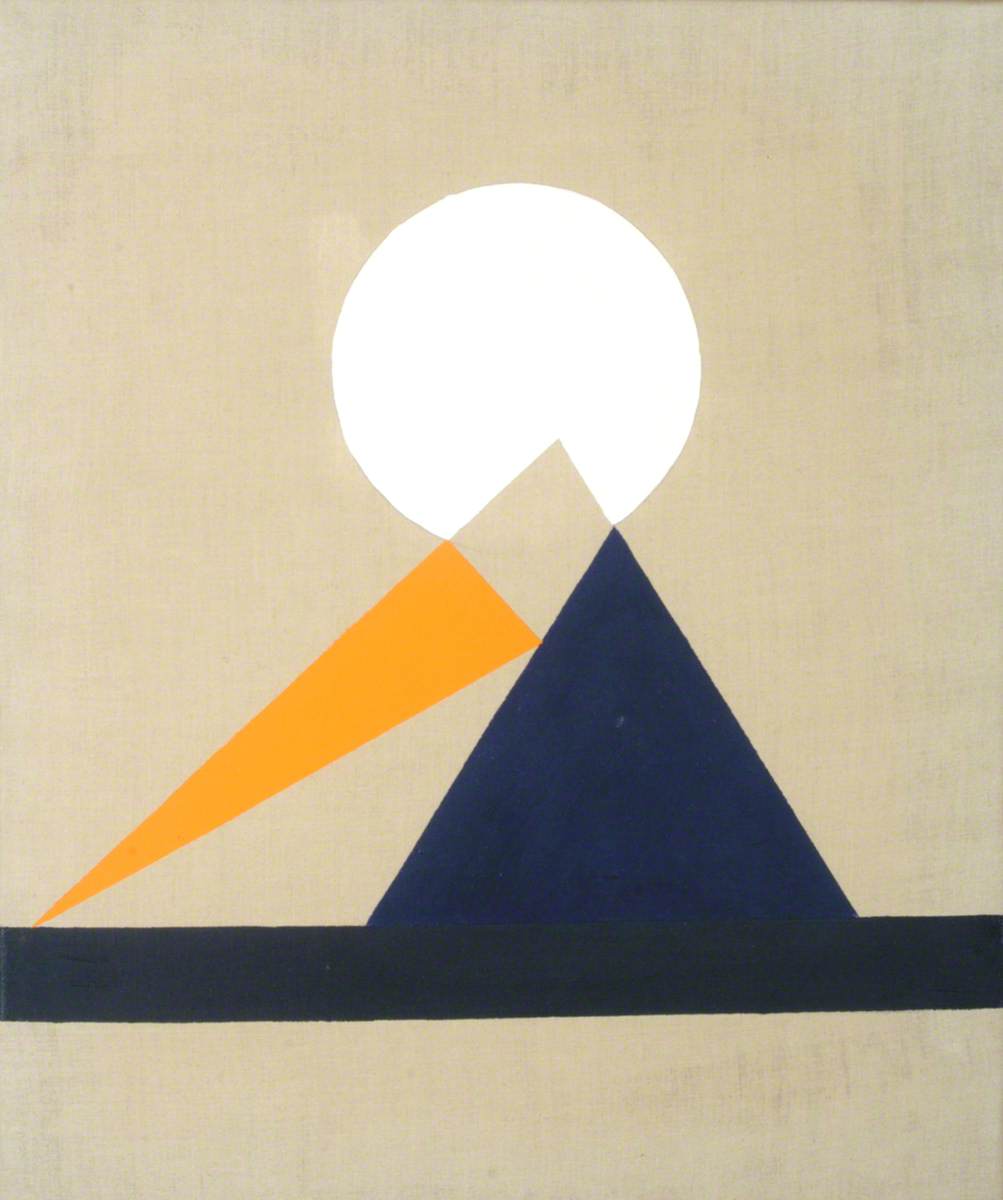The image is a detailed abstract art illustration in a portrait orientation. The background is a textured beige with vertical lines and gray streaks in the upper right corner. At the base of the image, a thick black horizontal line stretches across, grounding the composition. Resting atop this line and positioned slightly off-center to the right is a large, dark blue triangle. A thin gray diamond touches the peak of this triangle, adding a geometric accent. To the left of the blue triangle, slightly elevated, is a slim gold triangle that leans against it. Above these shapes is a large, white circular shape, reminiscent of a sun or moon, situated behind the peaks of the triangles. Additionally, an orange-yellow, elongated beak-like shape extends from the bottom left side of the blue triangle. The overall effect creates a stylized, almost pyramid-like structure against a minimalist backdrop, balancing simplicity with intricate detail.